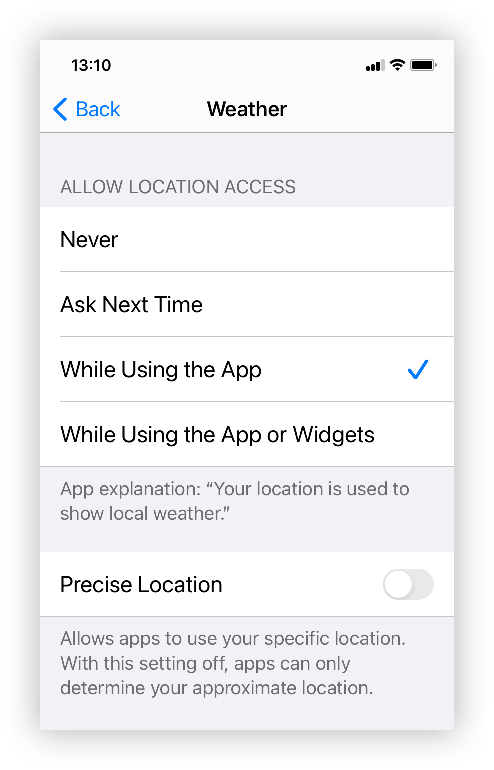The image depicts a smartphone interface, specifically focusing on the weather settings screen. At the top of the screen, the time is displayed as 13:10. In the right-hand corner, various status icons are visible, including the signal bars indicating internet connection, the Wi-Fi symbol, and the battery life indicator.

Directly below the status bar, there is a blue back button with an arrow, providing an option to return to the previous screen. The main section of the screen is titled "Weather" and prompts the user to "Allow location access," offering four choices: "Never," "Ask Next Time," "While Using the App," and "While Using the App or Widgets," with a check mark next to "While Using the App," indicating the currently selected option.

Further down, there is a note labeled "App Explanation," stating, "Your location is used to show local weather." Below this explanation, there's an option for "Precise Location," which can be toggled on or off. In the image, this setting is toggled off. The description beneath "Precise Location" explains, "Allows apps to use your specific location. With this setting off, apps can only determine your approximate location."